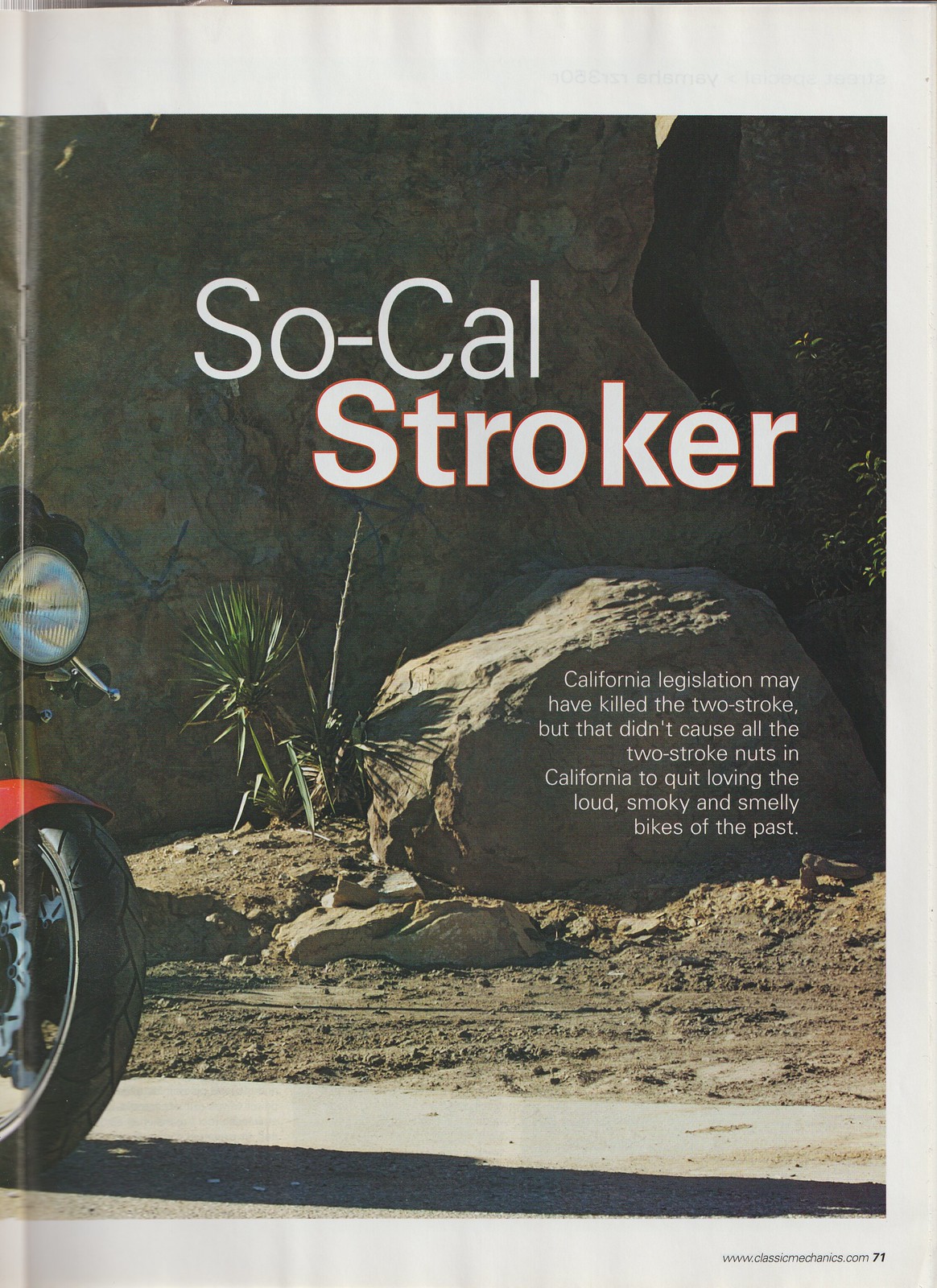This advertisement from a magazine, positioned on page 71 of www.classicmechanics.com, showcases a scenic desert landscape featuring a large rock outcrop and boulders, accented with sparse desert vegetation. In the foreground, the front wheel and light of a red-colored motorcycle protrude from the left edge, partially folded over, casting a long shadow on the road below. Central to the image, bold white text outlined in red reads "So-Cal Stroker." Additionally, smaller white text overlaid on a smaller rock to the right states, "California legislation may have killed the two-stroke, but it didn't cause all the two-stroke nuts in California to quit loving the loud, smoky, and smelly bikes of the past." This visually striking spread hints at an event or feature that celebrates the enduring passion for two-stroke motorcycles despite regulatory challenges.